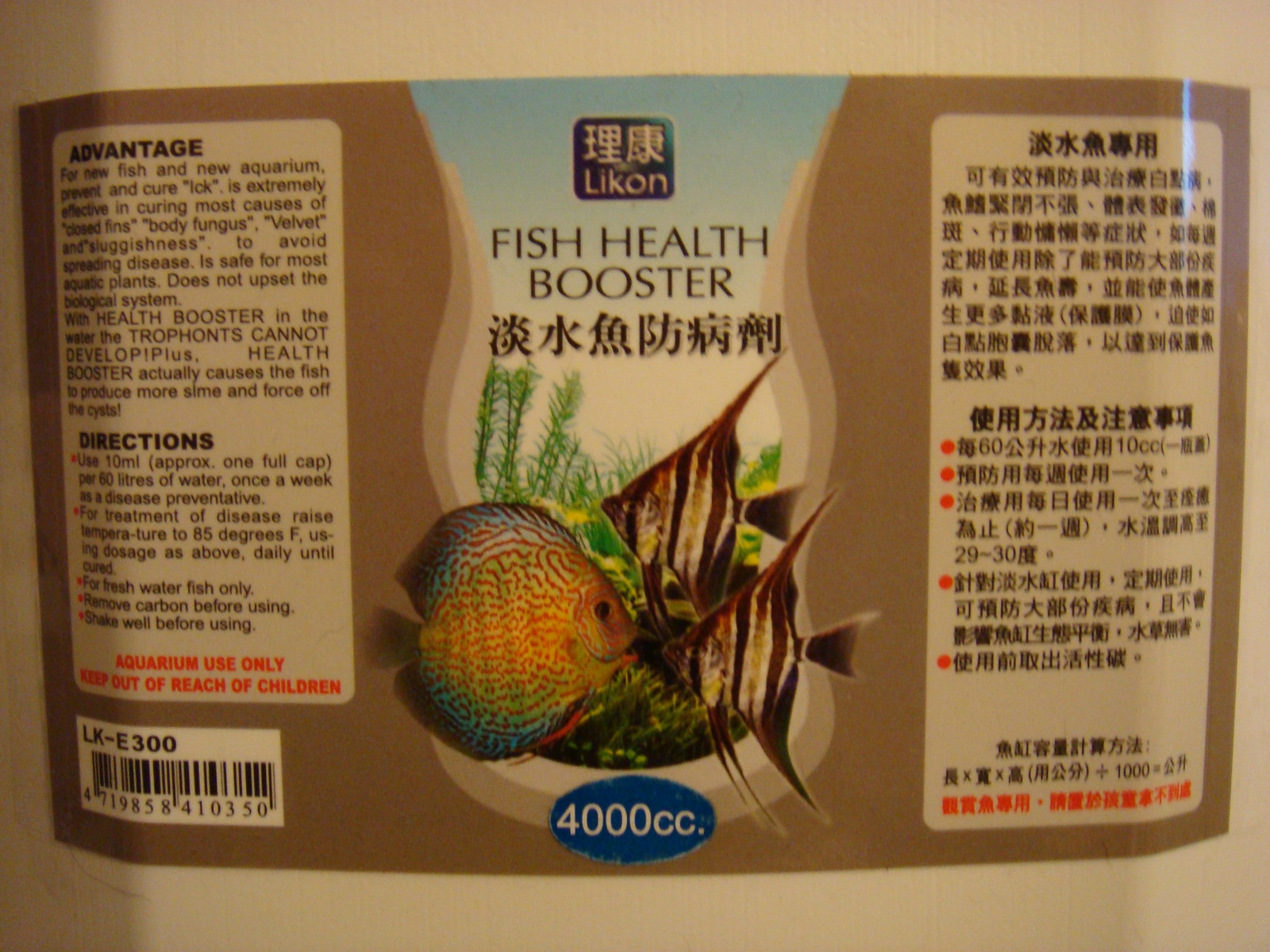The label, likely for a fish health supplement on a curving brown bottle, features a central, colorful image of three fish. The largest fish is vibrant with hues of yellow and blue heading right, flanked by two leftward-swimming striped fish with brown and yellow, pointy fins. The background appears tannish at the top and bottom, giving an aquarium-like impression with some visible plants. 

Prominently, the text "Fish Health Booster" is centered at the top, under the logo "Lykon" with Chinese characters framed by symbols. Below the central image, there's a blue oval indicating "4,000 cc." To the right, the text is in Chinese, accompanied by small orange dots. The left side, in English, starts with "Advantage," detailing its benefits for new aquaria. It prevents and cures various fish ailments such as ick, body fungus, and velvet, without disturbing the biological system. Directions are listed below, accompanied by orange dots, emphasizing raising the temperature for effective use and other instructions. At the bottom, in bold orange letters, it warns, "Aquarium use only. Keep out of reach of children," next to a UPC label in the bottom left corner.